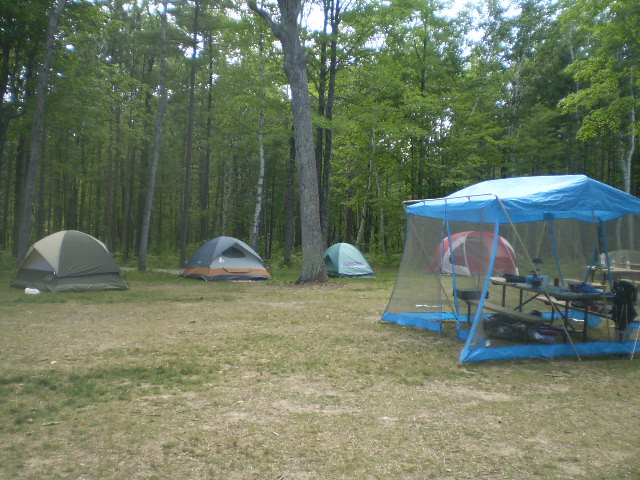The image captures a serene campground situated in a dense forest with tall trees and lush, green foliage. The forest floor is covered with patchy, semi-balding grass that appears brown in some areas. At the right center of the photograph, there is a screen tent with a blue top and bottom, encasing a picnic table and various cooking equipment. In the background, four dome tents are lined up in front of the forest tree line. From left to right, the tents are olive and tan, green and orange, light blue, and finally, red and white. The scene is devoid of people, buildings, or vehicles and appears to be taken during the day under a cloudy sky. The colors in the image include a mix of green, brown, tan, gray, light blue, orange, red, and white, giving it a vibrant yet natural feel.